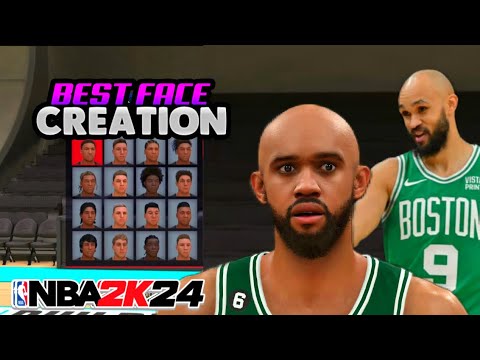A detailed screenshot from the video game NBA 2K24 is shown. The game’s title, 'NBA 2K24,' with '2K' highlighted in red, appears near the bottom-left corner alongside the NBA logo. At the top of the screenshot, the title 'Best Face Creation' is prominently displayed, with 'Best Face' in purple and 'Creation' in larger gray letters. The main section features a four-by-four grid showcasing various face options, with the top-left face visibly highlighted in red.

To the right of this grid, there is a depiction of a basketball player in two different poses. The closer perspective reveals the player with his mouth open, sporting a beard and wearing a green Boston jersey labeled with the number 6. The further perspective shows the same player seemingly engaged in conversation, wearing the number 9 Boston jersey. Both jerseys are green with the 'Boston' name and have a visible Nike logo. The background setting includes a stadium or auditorium, evident from the visible seating and a section of the basketball court floor.